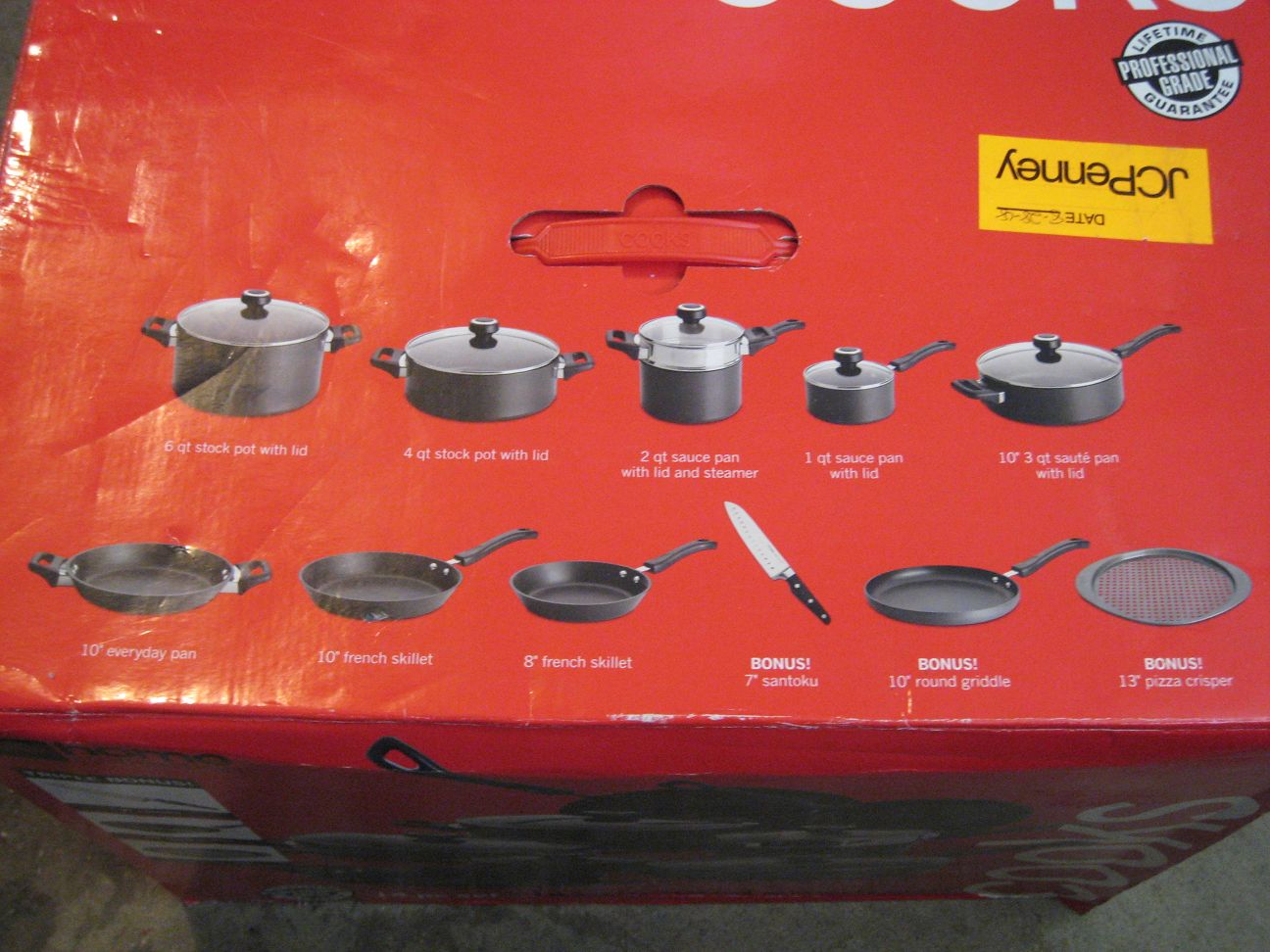This image features a large, red JCPenney box adorned with a bold, yellow and black "JCPenney" label prominently on top, along with a "Lifetime Guarantee Professional Grade" badge in the upper right-hand corner. The box serves as a container for an extensive collection of kitchen cookware and utensils. The detailed images on the box illustrate its contents, including a six-quart stock pot with a glass lid, a four-quart stock pot with a glass lid, a two-quart saucepan with a glass lid and steamer, a one-quart saucepan with lid, a three-quart saucepan with lid, an eight-inch French skillet, a ten-inch French skillet, a ten-inch everyday pan, a pizza crisper, a ten-inch round griddle, and a seven-inch santoku knife. The red box features a sturdy handle indicating its heavy weight and appears to have been opened and resealed at some point.